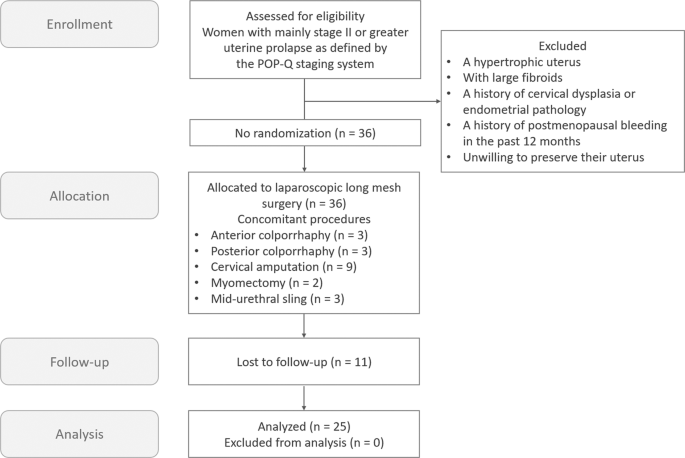The image depicts a detailed flowchart diagram resembling a PowerPoint slide, illustrating different stages of a clinical trial process for women with mainly stage 2 or greater uterine prolapse, as defined by the POPQ staging system. The left-hand column comprises sections labeled "Enrollment," "Allocation," "Follow-Up," and "Analysis," with corresponding detailed descriptions to the right of each label. In the "Enrollment" section, it specifies that participants were assessed for eligibility, with inclusion criteria focusing on women predominantly in stage 2 or greater uterine prolapse. It notes that 36 participants were enrolled without randomization. The flowchart highlights excluded subjects, specifying reasons such as hypertrophic uteri with large fibroids and a history of cervical dysplasia or endometrial pathology. The diagram flows systematically with arrows and rectangles guiding from initial assessment through allocation to follow-up and final analysis.